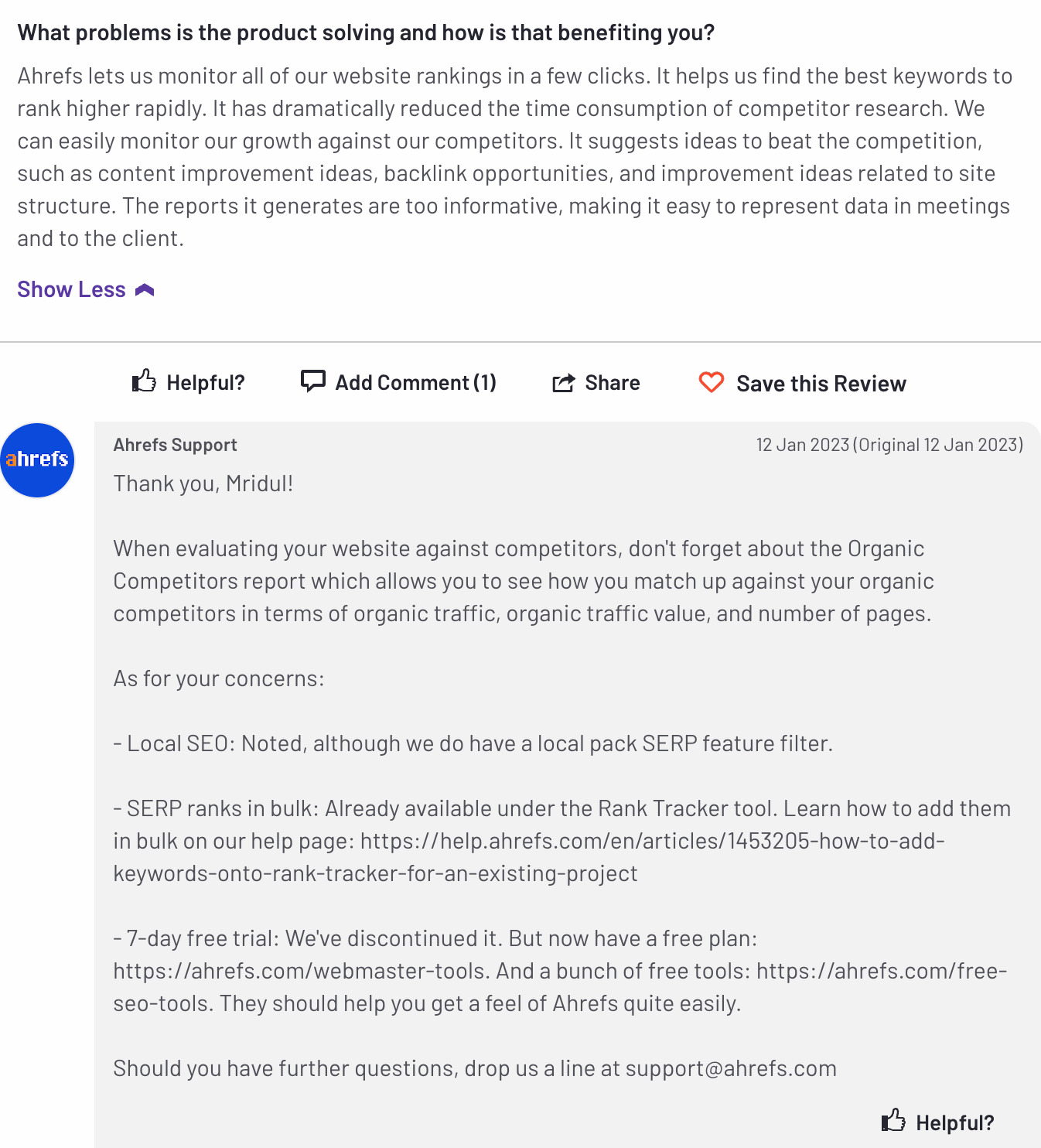The image depicts a review section of a website. Across the top, a question is displayed in bold black font: "What problems is the product solving and how is that benefitting you?" Below this, a user's review is shown in a lighter shade of black font, responding to the question.

On the left side, there's a clickable "Show less" link in purple, accompanied by an upward-pointing arrow. A thin, light blue line separates this portion of the image from the rest of the content.

Directly beneath the line, there are several clickable icons – "Helpful," "Add Comment," "Share," and "Save this Review" – providing options for user interaction.

Further down, a company representative has replied to the review. This response is marked with a blue circle featuring the company's initials. The representative thanks the reviewer for their feedback and addresses some of their concerns. Their reply is enclosed within a light blue box. In the bottom right corner of the response, there is an option to mark the reply as helpful.